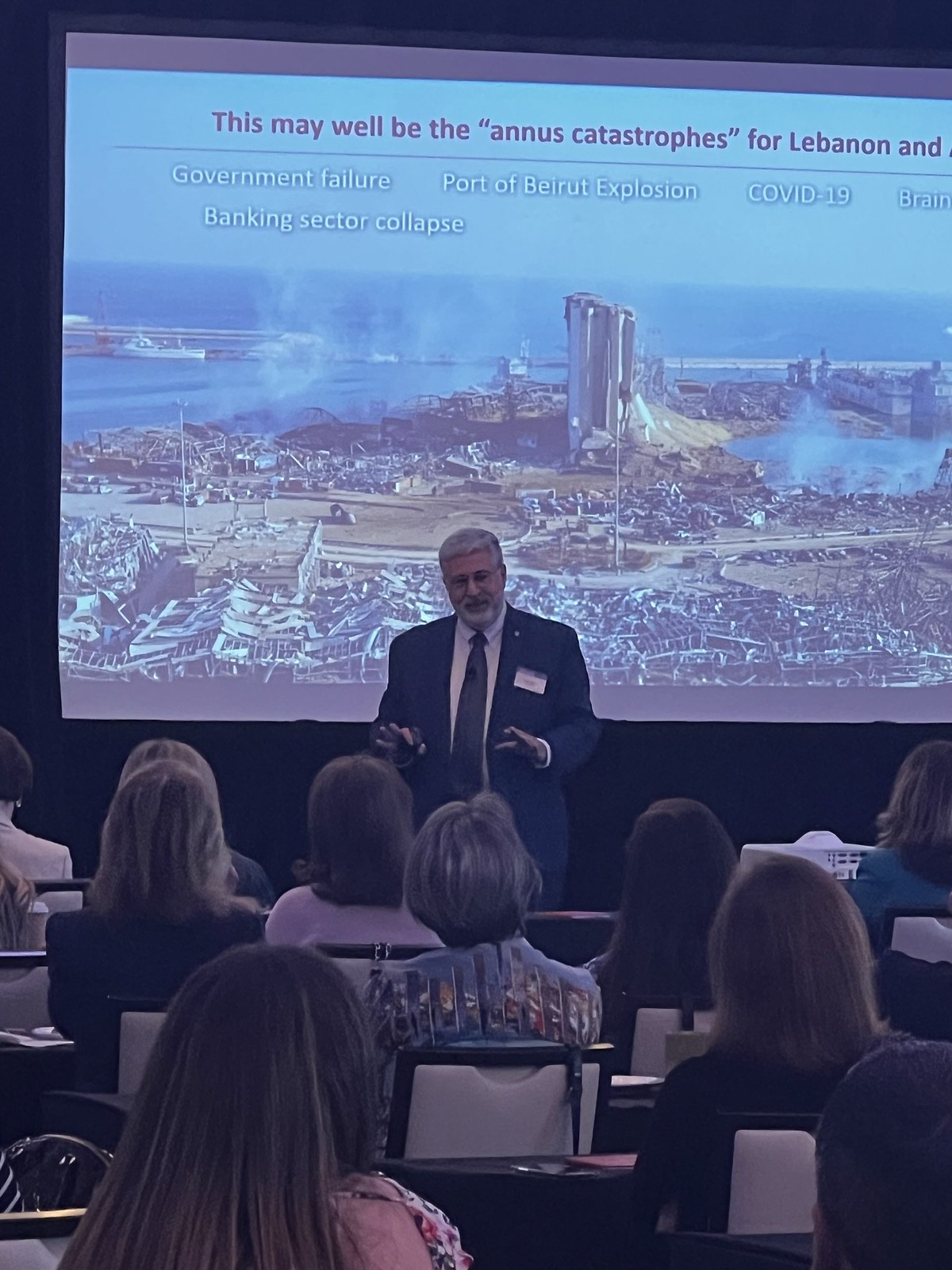An indoor photograph captures a semi-dark room where approximately ten women are seated in white chairs with black metal frames in front of small black desks, closely listening to an older white man presenting on stage. The man, wearing a black suit, black tie, and a white button-up shirt, with white hair and a beard, gestures with his hands while speaking. He also has glasses and a name tag. Behind him, a large projection screen displays an image of a devastated coastal city with a towering building amidst widespread destruction. The screen headlines with "This May Well Be the Anas Catastrophes for Lebanon" and enumerates contributing factors to Lebanon’s suffering in white text: government failure, the Port of Beirut explosion, COVID-19, and a banking sector collapse. The attentive audience, their purses draped over chair backs, stare directly at the speaker, absorbing the dire details of the presentation.